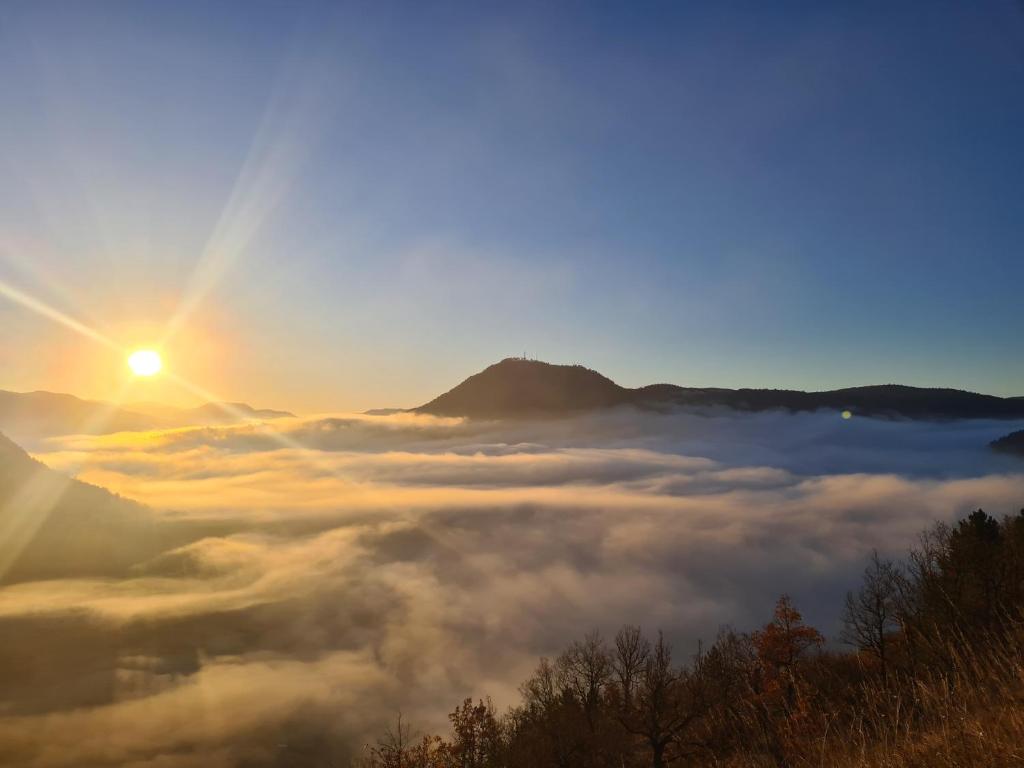This captivating real-life photograph, captured from a high vantage point atop a mountain, exquisitely showcases a breathtaking sunset. The sky, predominantly clear with a few scattered clouds, features a brilliant, yellow-orange sun situated towards the top left. Radiating from the sun are four distinct beams, or God rays, forming a cross-like pattern that enhances the natural beauty of the scene.

In the foreground, the rugged mountain slope is densely covered with winter foliage, characterized by brown hues among trees and brush. Descending down from this mountaintop, the setting reveals an expansive valley cloaked in a thick, white blanket of fog, giving a mystical, smoky appearance. Emerging from this ethereal fog are several mountain peaks, most notably a prominent one centrally positioned in the background, enveloped by the mist. To the left, a smaller mountain range trails off with another range visible above it. The scene, devoid of any human presence or text, captures the serene and majestic essence of nature from a lofty perspective, with elements of blue sky, orange sunlight, and the contrasting whites and grays of the fog and distant snow.